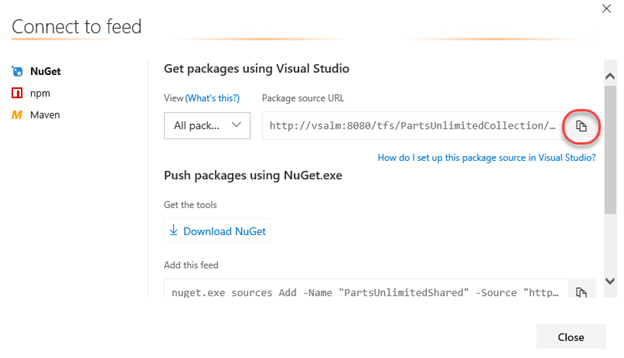The image features a white background predominantly at the top, with the phrase "Connect to feed" displayed alongside a broken red line. Below this, the terms "Nugget," "RPM," and "Maven" are listed. A prominent blue box states, "Get packages using Visual Studio," accompanied by options that include "View," "What's this," and an additional box labeled "All pack" with a downward-facing arrow, likely indicating a dropdown menu.

Further down, there is a "Package source URL" field displaying an HTTP address. Adjacent to this, an icon depicting two overlapping papers is visible with the text, "How do I set up this package source in Visual Studio?" On the right side of the page, a long, light-blue scrollbar is present with both up and down arrows.

Additional instructions read, "Push packages using NuGet.exe" and "Get the tools." Underneath, a box with another downward arrow is labeled "Download NuGet." There is a section with the command, "NuGet.x.sources add name," followed by "part, sun, LL, or Limited, Shared," and "source" with another HTTP link.

A small square icon, possibly representing buildings or a related symbol, appears next to the mentioned commands. The image also includes a "Close" button at the bottom, potentially to exit or complete the setup process.

Overall, the detailed visual guide provides clear instructions and interface elements relevant to connecting and configuring package sources and tools within Visual Studio, specifically focusing on NuGet package management.